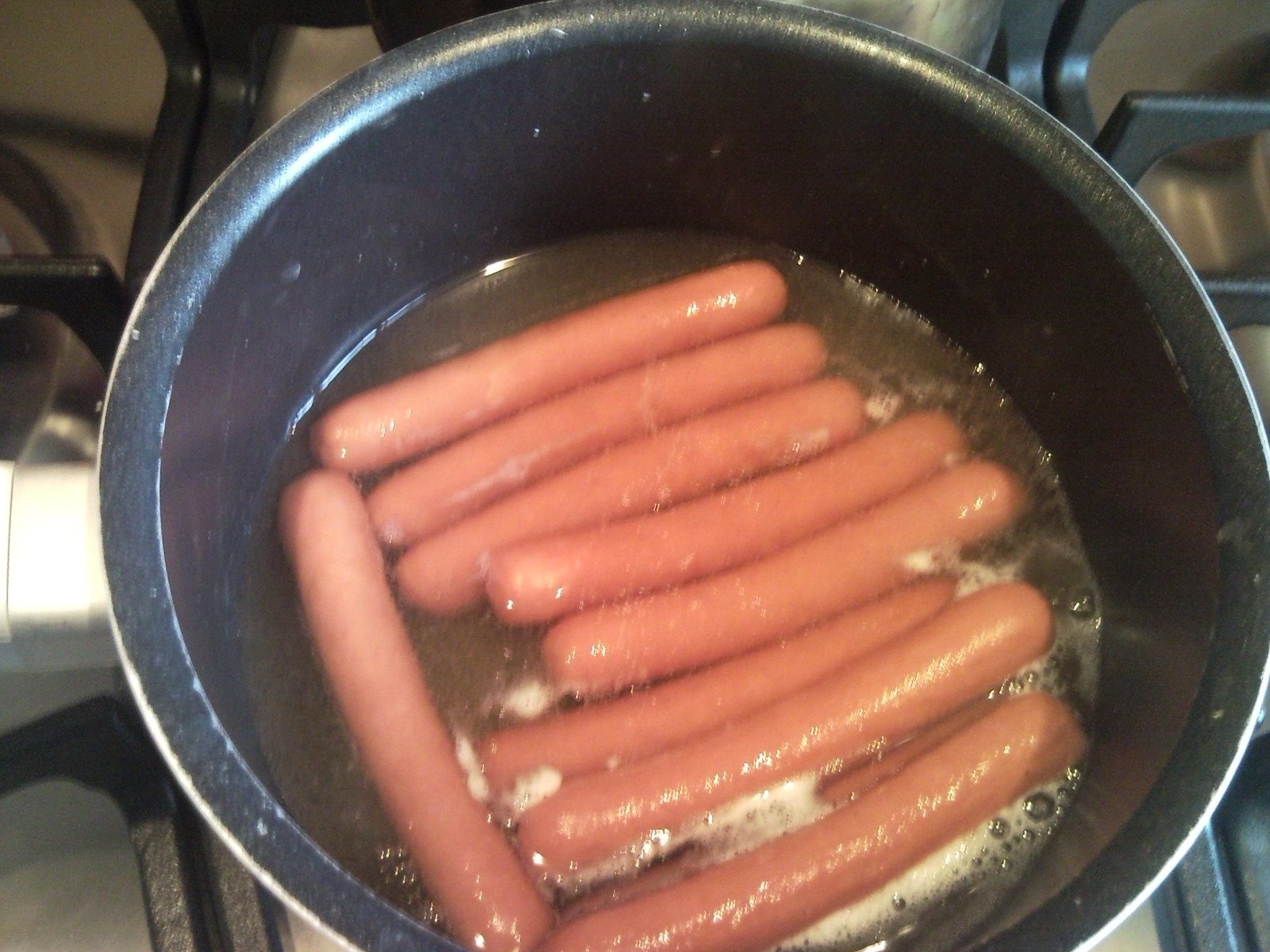This top-down photograph captures a black, worn, nonstick pot with a thin white rim, filled with ten hot dogs boiling in a foamy, brownish water that appears somewhat rancid. The hot dogs are mostly submerged, save for a couple near the bottom resting atop others and protruding from the water. The water is bubbling lightly, and a layer of white foam clings to the hot dogs’ surfaces, adding to their unappealing appearance. In the background, partially visible black metal burners hint at the gas stovetop location, while another pot is faintly discernible near the top of the image. The scene suggests a grimy kitchen environment, emphasizing the neglected condition of the cooking vessel and overall setup.